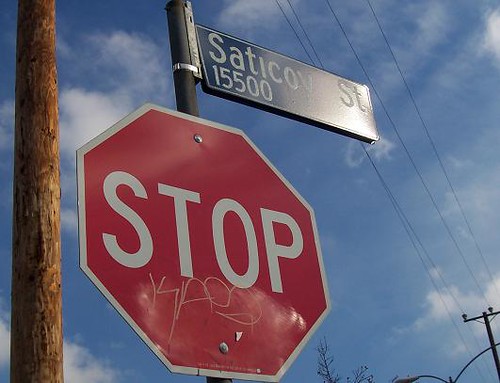This photograph, taken on a bright, sunny day, captures a street scene dominated by a clear blue sky. On the left side of the image stands a wooden power line pole extending upward. Adjacent to the pole, a stop sign on a metal pole marks the intersection. Above the stop sign, a green street sign displays "Satico Street 15500" in white letters. The stop sign itself features a red background with white letters and trim, marred by squiggly graffiti reading "K-A-O-S" near its bottom, secured by a nail. Overhead, power lines crisscross the sky, while the top right corner of the photo hints at the presence of a street light, starting to come into view.